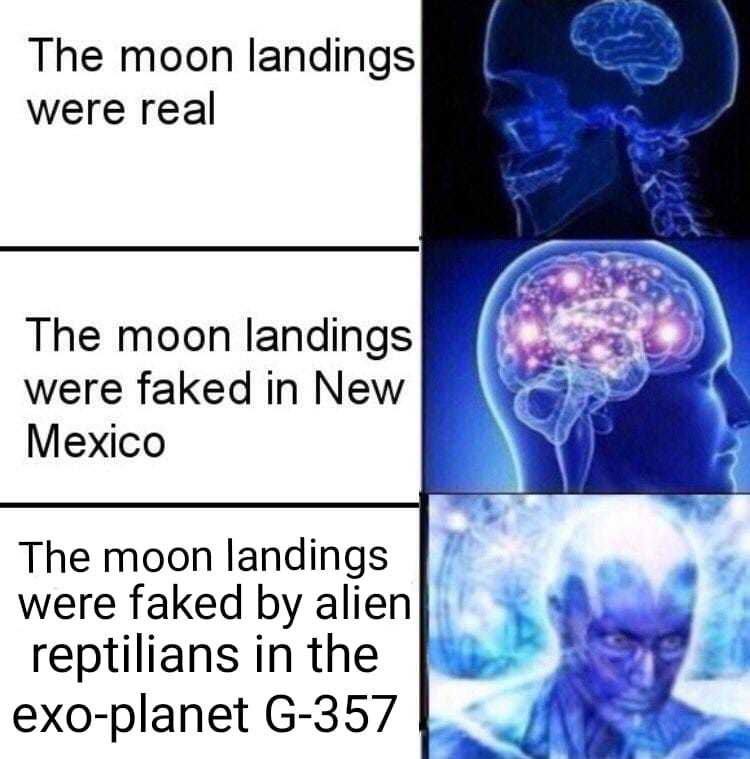The meme consists of three vertically aligned sections, each containing an image of a humanoid head against a dark blue and black background. On the right-hand side, the top image depicts an X-ray-like head with a very small brain. The middle image features an artistic rendering of an illuminated brain with intricate lighting effects, showcasing increased brain activity. The bottom image is of a more abstract, almost skinless blue figure, emanating light and energy from its head. Each section has corresponding humorous text on the left: "The moon landings were real" for the X-ray head, "The moon landings were faked in New Mexico" for the illuminated brain, and "The moon landings were faked by alien reptilians in the exoplanet G357" for the abstract figure. The meme humorously escalates conspiracy theories about the moon landings, visually represented by increasingly complex and energetic brain imagery.